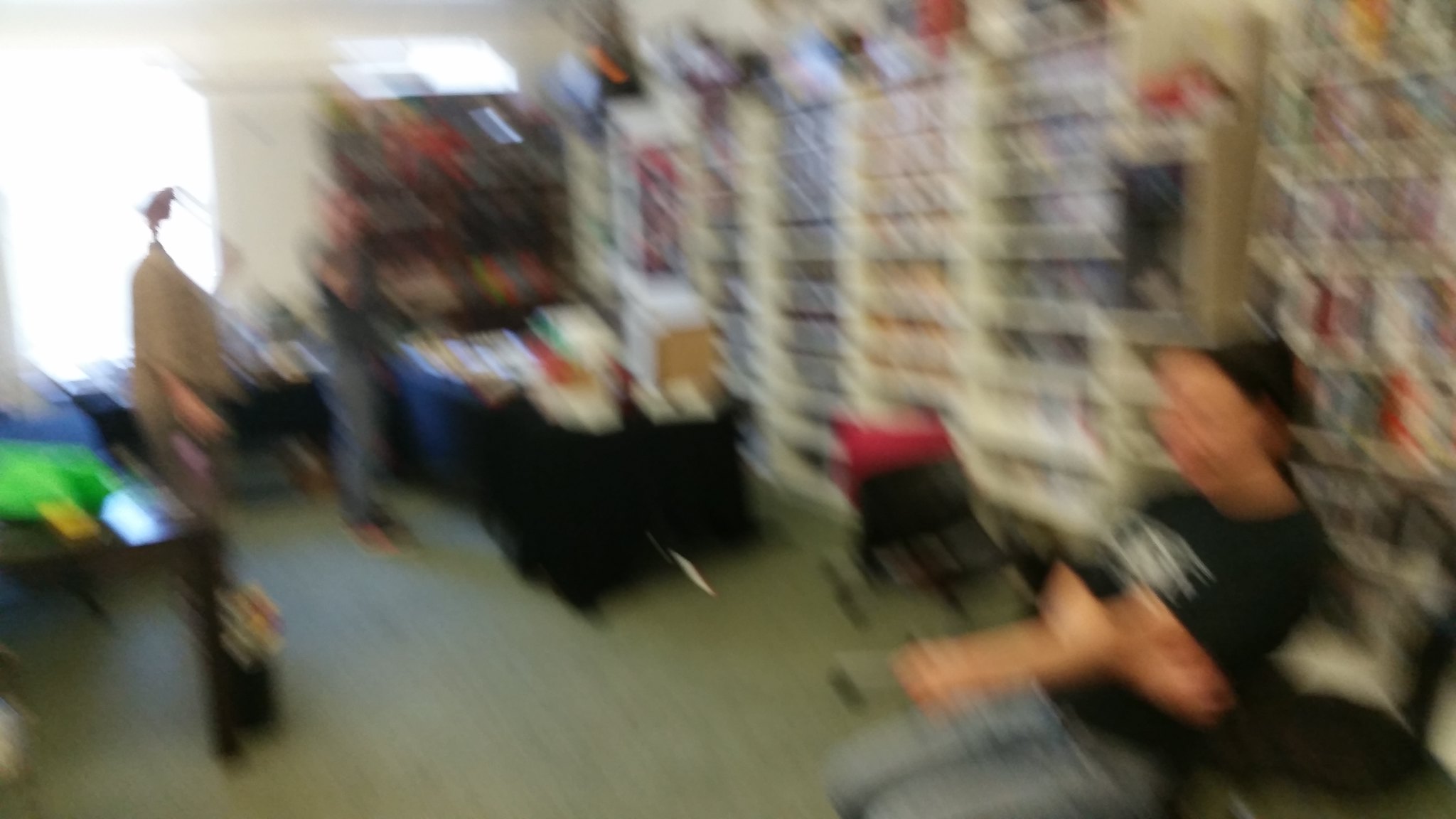In this blurry photograph of what appears to be a shop, the main focal point is a bright window on the top left that obscures the face of a woman standing nearby. The scene includes multiple elements: towards the back are two people, one in a khaki suit and another in a gray shirt with blue jeans. In the near view, a woman in a black shirt with white symbols, blue jeans, and possibly a black hat is seated in a chair, with her hair tied back in a ponytail; she might also be wearing glasses.

The shop features a variety of displays and shelves: on the right-hand wall, an array of dark-colored items arranged in rows, possibly fabric samples, underwear, or books. Above these samples, there may be flags. Centrally, there are black and blue stands capped with indeterminate items. A black display table towards the back holds a white pile of some sort, and a brown table next to it supports green and blue packaged items.

Additional shelving includes a white shelf on the back wall stocked with assorted items that could be books or collectibles, alongside a brown wooden shelf. The floor appears to be a grayish carpet. Overall, the image is chaotic yet detailed with various objects and individuals contributing to the bustling atmosphere of the shop.